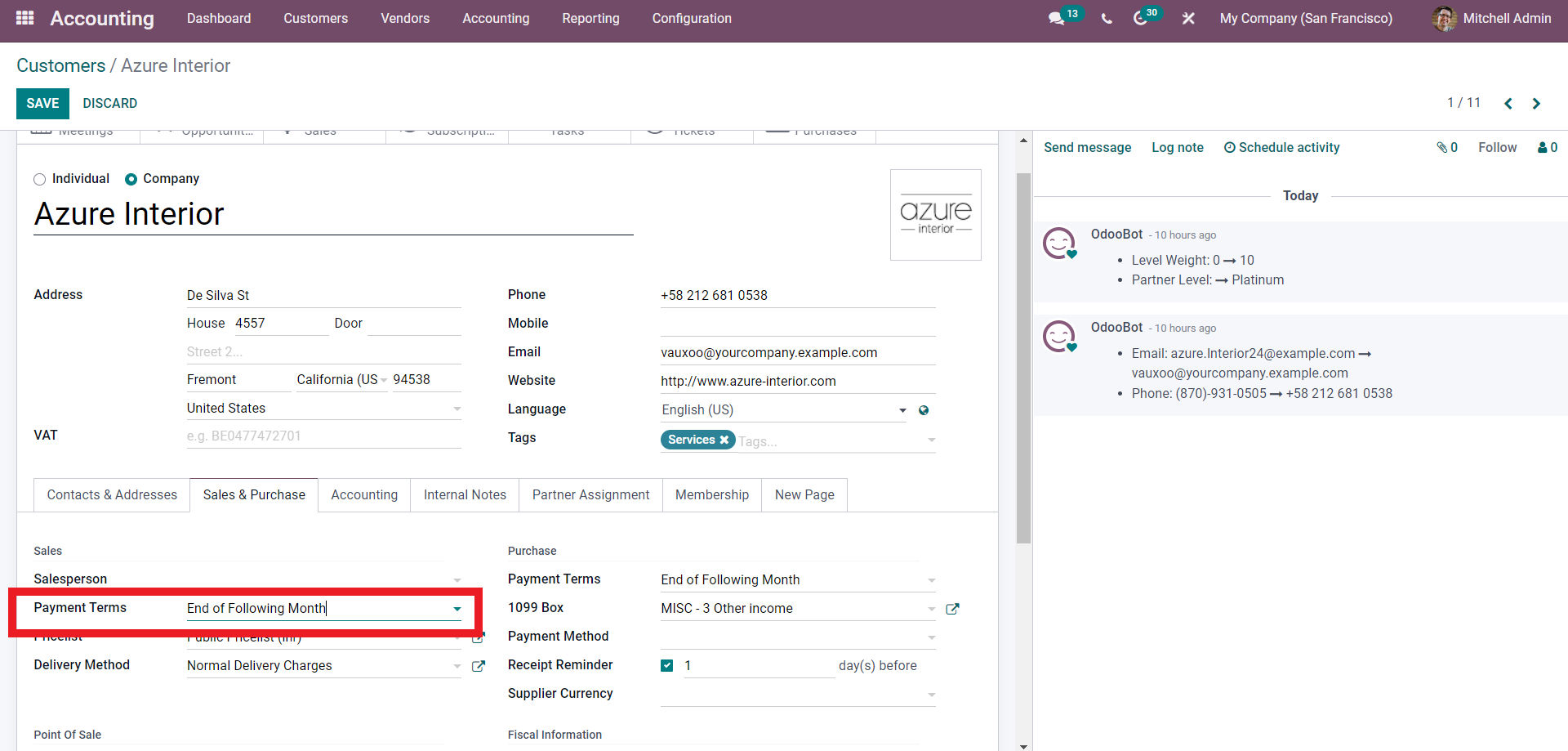The image is a screenshot of a computer screen displaying an accounting software interface. At the top of the screen, there is a horizontal, purplish-burgundy rectangle spanning the width of the display, with the word "Accounting" prominently featured in white text.

Beneath the main heading, there is a navigation menu in smaller white print, listing several options: "Dashboard," "Customers," "Vendors," "Accounting," "Reporting," and "Configuration." On the right side of this top section, there are several icons: two speech bubbles with the number 13 in a green circle, a phone icon, and a clock icon with the number 30 in another green circle. An 'X' icon is also visible in this area.

Just below the main navigation, the screen displays the text "My Company, San Francisco" alongside a profile picture, labeled "Mitchell Admin."

Further down, there is a section titled "Customers / Azure Interior." Within this section, there is a green "Save" button and a "Discard" button, the latter of which is simply highlighted in green text.

The screen continues with more details about "Azure Interior," including fields for the address and VAT information. A significant detail is the section labeled "Payment Terms," specifically highlighted with a red rectangle. The payment terms are stated as "End of Following Month."